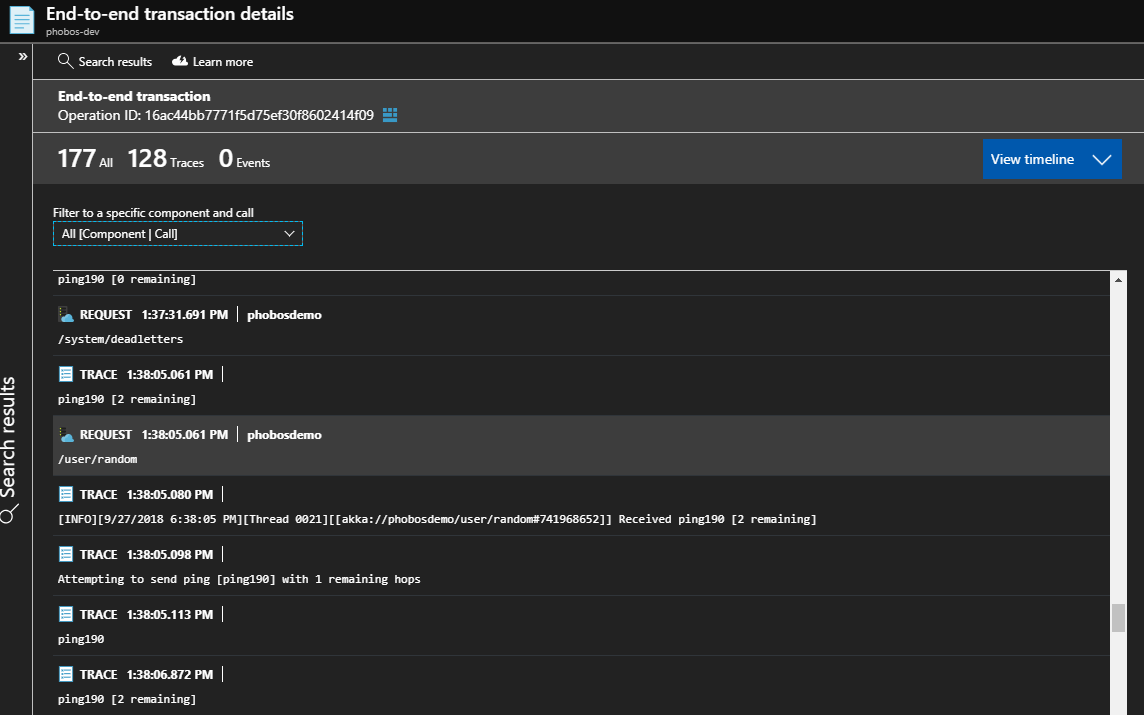The image predominantly features a dark background, intensifying the contrast with the lighter elements in the foreground. In the top-left corner, a light blue icon resembling a piece of paper, bordered by a darker blue edge, stands out. Adjacent to this icon is white text that reads "End-to-End Transaction Details."

Directly beneath this title, there's a long, rectangular tab, reminiscent of an internet browser tab. Continuing downward, beneath the earlier white text, appears light gray text indicating "Search Results." To its immediate right, white text prompts the user to "Learn More."

The image further exhibits two elongated horizontal rectangles, both in light gray, containing white textual information. The first rectangle displays "End-to-End Transaction" followed by "Operation ID" alongside an extensive string of text and numbers. The second rectangle provides numerical information in white: "177 All," "128 Traces," and "0 Events."

Below these boxes, an array of white text entries is visible. The first entry reads "Request," followed by "/System/Dead Letters." Subsequent lines of text include "Trace," followed by additional "Request" and several rows of "Trace." 

On the image's top-right corner, a blue rectangular button displays the white text "View Timeline." Along the left side, a vertical rectangular box in darker gray features the text "Search Results" in white. Finally, the bottom-right corner of the image includes a portion of a light gray scroll bar.